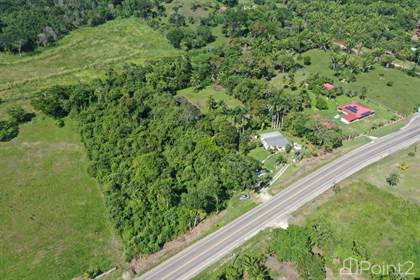This aerial photograph showcases an expansive plot of land, visually divided between lush greenery and open fields. Dominating the landscape are dense clusters of trees and shrubbery interspersed with cleared grassy areas. A two-lane roadway cuts through the lower right section of the photo, labeled "Point 2," adding a sense of scale and structure to the scene. 

Adjacent to this road is a noticeable red-roofed building. Nearby, another smaller structure lies diagonally towards the center, while a larger, white building with a gray roof is positioned further alongside. On the left side of the image, the open field is free from any significant vegetation. 

In the background, you can discern a small roofed area, presumably part of a house, hinting at residential occupation within this plot. Neighboring this property, another distinct residence with a pink roof, along with a secondary pink-roofed shelter, stands out, enveloped by trees and greenery. The aerial view underscores the serene and spacious layout of the acreage, bathed in clear daylight, with woods framing the entire expanse.